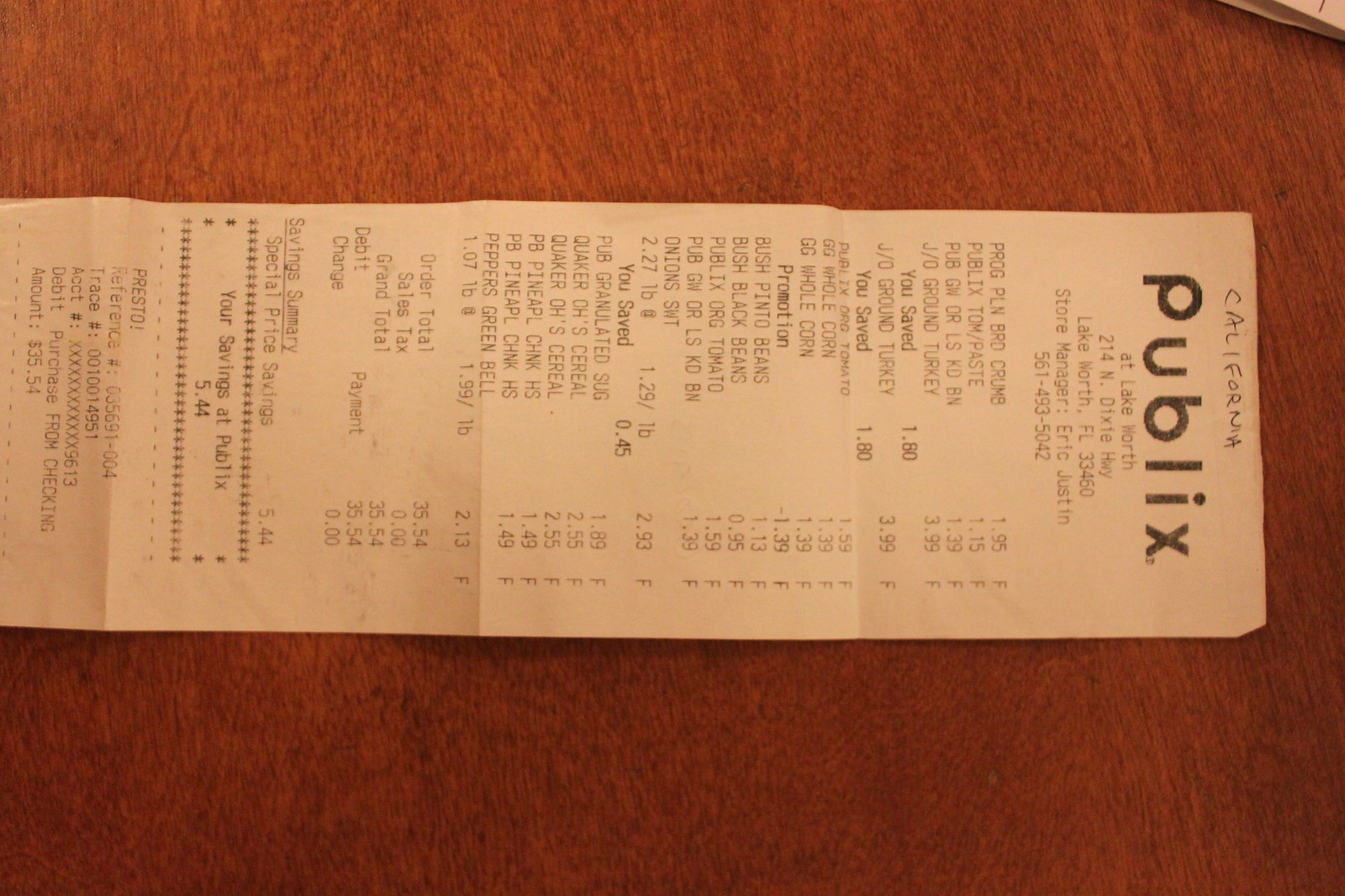The photograph depicts a receipt placed on a vibrant red-orange wooden surface, accented with lighter colored and black veining that adds texture and depth to the wood. The receipt is positioned face up, viewed from a sideways angle such that the text at the top, "Publix," appears vertically with each letter stacked beneath the previous one. Beneath the store name, several rows of black text are centered on the receipt, detailing the transaction. On the left side of the receipt, perpendicular to our view, is a list of purchased items. Their corresponding prices are aligned to the right, translating to the bottom edge of the receipt in this perspective. Below the itemized section, the total and tax amounts are listed. Near the bottom, a row of asterisks brackets a segment of text, with another row of asterisks framing the section below. Further black writing is found at the very base of the receipt, completing the document's detailed record of the purchase.